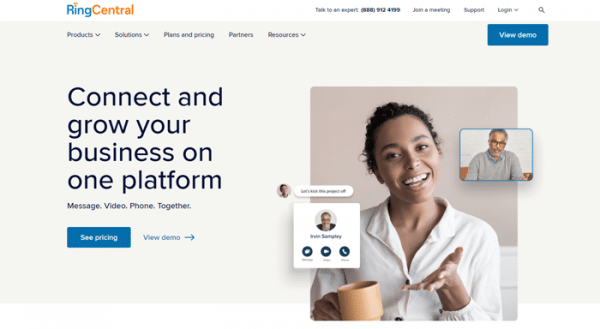The homepage of RingCentral features a sleek design with intuitive navigation. At the top, a series of tabs include "Products" (with a drop-down menu), "Solutions" (with a drop-down menu), "Plans & Policies," "Pricing," "Partners," and "Resources" (with a drop-down menu). Dominating the page is a central message reading, "Connect and grow your business on one platform: message, video, phone together," emphasized in bold text.

Two prominent blue buttons, "View Demo" and "See Pricing," catch the viewer's eye, inviting them to explore further. Below, a preview of the demo is showcased, depicting a video conversation between a woman and a man. The woman, likely in her late 20s to early 30s, is biracial and dressed in a casual off-white blouse. She holds a mug in her right hand and gestures animatedly with her left. On the other side of the video call is an African American man in his 50s, sporting a gray shirt and prescription glasses, with visible gray hair. This visual effectively highlights the platform's video communication capabilities, suggesting its seamless integration for business interactions.